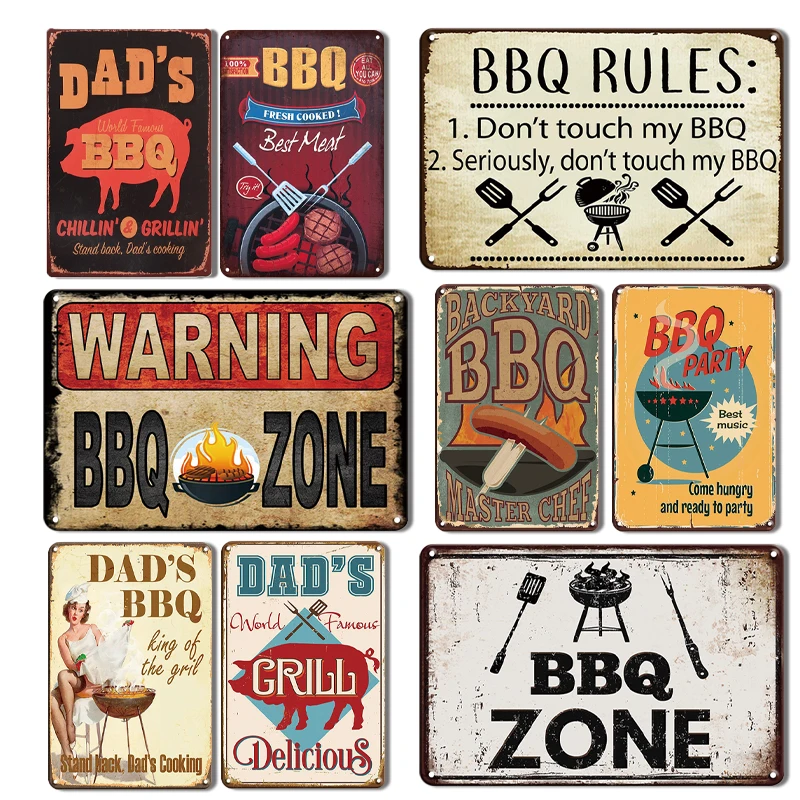The image showcases a collage of nine vintage-style barbecue signs, each with a rustic and worn metal aesthetic. The signs feature a variety of colorful designs and humorous messages. 

- The top-left sign says "Dad's BBQ" in bold text on a pinkish coral pig silhouette, accompanied by the phrase "Chillin' and Grillin'".
- Next to it, a sign displays a grill with sausages and hamburgers, reading "BBQ Fresh Cooked, Best Meat".
- Further right, a sign humorously outlines "BBQ Rules: 1. Don't Touch My BBQ 2. Seriously, Don't Touch My BBQ".
- Below these, a bright red warning sign states "BBQ Zone", mimicking a safety warning.
- Another sign near the center reads "BBQ Backyard BBQ Master Chef".
- On the far-right, a festive sign announces a "BBQ Party" with a grill illustration and the invitation to "Come Hungry and Ready to Party".
- Lower down, another sign warns again with "BBQ Zone" in bold red.
- Additional signs include "Dad's BBQ King of the Grill" with retro imagery and "Dad's Grill World Famous, Delicious".

Each sign blends colorful illustrations of pigs, grills, and barbecue tools, emphasizing a fun, nostalgic, and celebratory barbecue theme perfect for home decor.